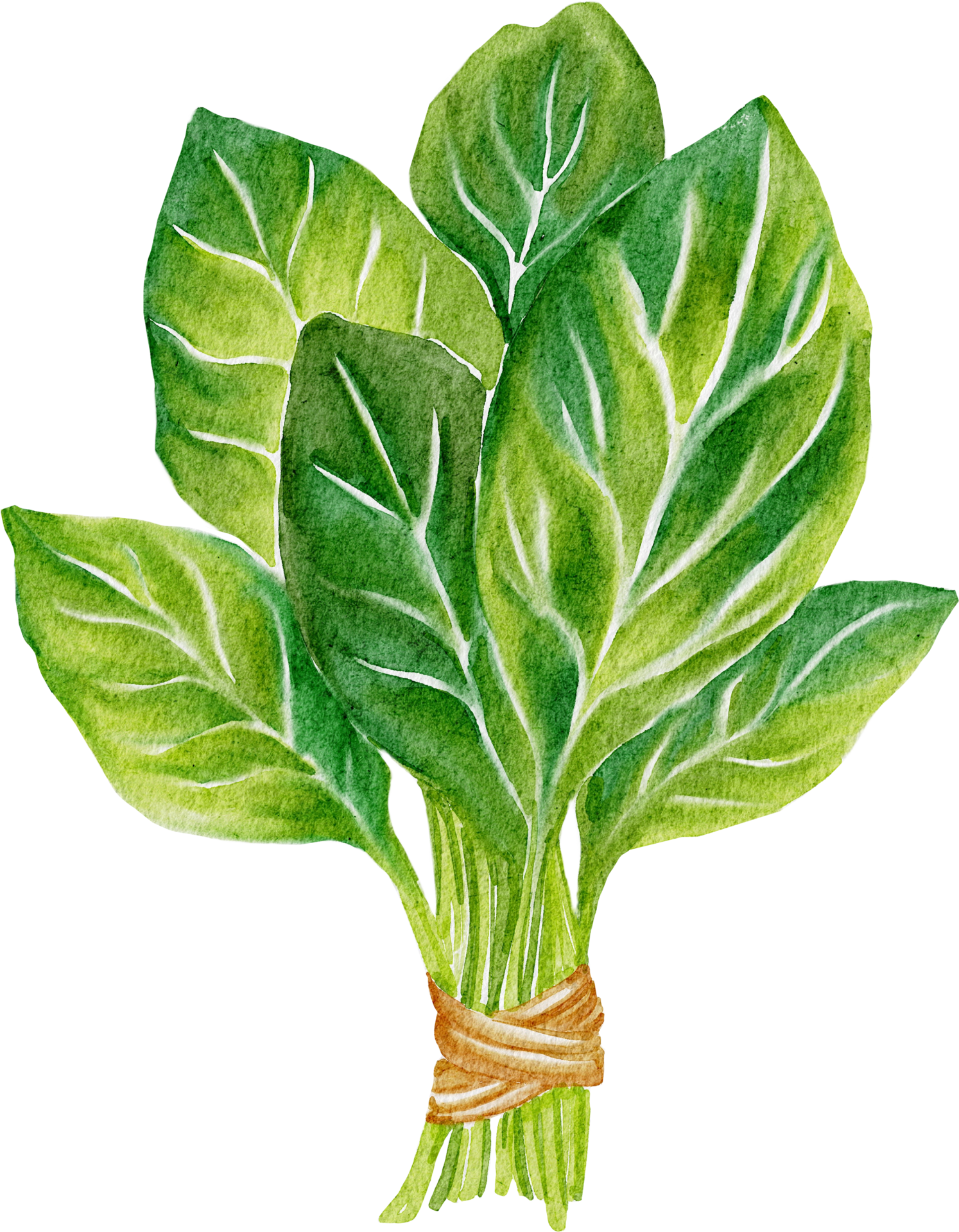This image is a detailed, stylized drawing of a bunch of six large green leaves, likely basil or spinach, intricately bound together at the stems with a double-crisscrossed brown twine. The leaves are depicted in various shades of green, accented with detailed white veins that run through them, adding texture and depth. The twine has a rust-brown hue with highlighted white accents, and the artwork appears to be created using watercolors or pastels, giving it a soft, hand-drawn appearance. The background is white and transparent, focusing all attention on the vividly illustrated foliage. This artistic piece could easily fit as decor in a restaurant, hotel, or someone's kitchen.